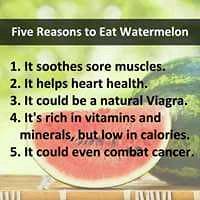The image is a small, square-format color photograph with a graphical overlay, creating an infographic. The background is a blurry, out-of-focus green, resembling trees or leafy vegetation, suggesting an outdoor setting with plenty of natural light filtering through. 

In the foreground, on a brown wooden table that could be a picnic table, there is a slice of watermelon positioned near the center bottom of the image. The slice is shown in profile, revealing its vibrant red interior, a cream-colored rind, and a dark green outer skin. Just behind the slice, towards the right, there is a partially visible whole watermelon.

A black banner stretches across the top of the image with white text that reads, "Five Reasons to Eat Watermelon." Below this banner, and also partially overlaid on the watermelon slice, the reasons are listed in black text:
1. It soothes sore muscles.
2. It helps heart health.
3. It could be a natural Viagra.
4. It is rich in vitamins and minerals but low in calories.
5. It could even combat cancer.

This detailed and realistic representation combines photographic elements with text to deliver a visually appealing and informative health-related message.